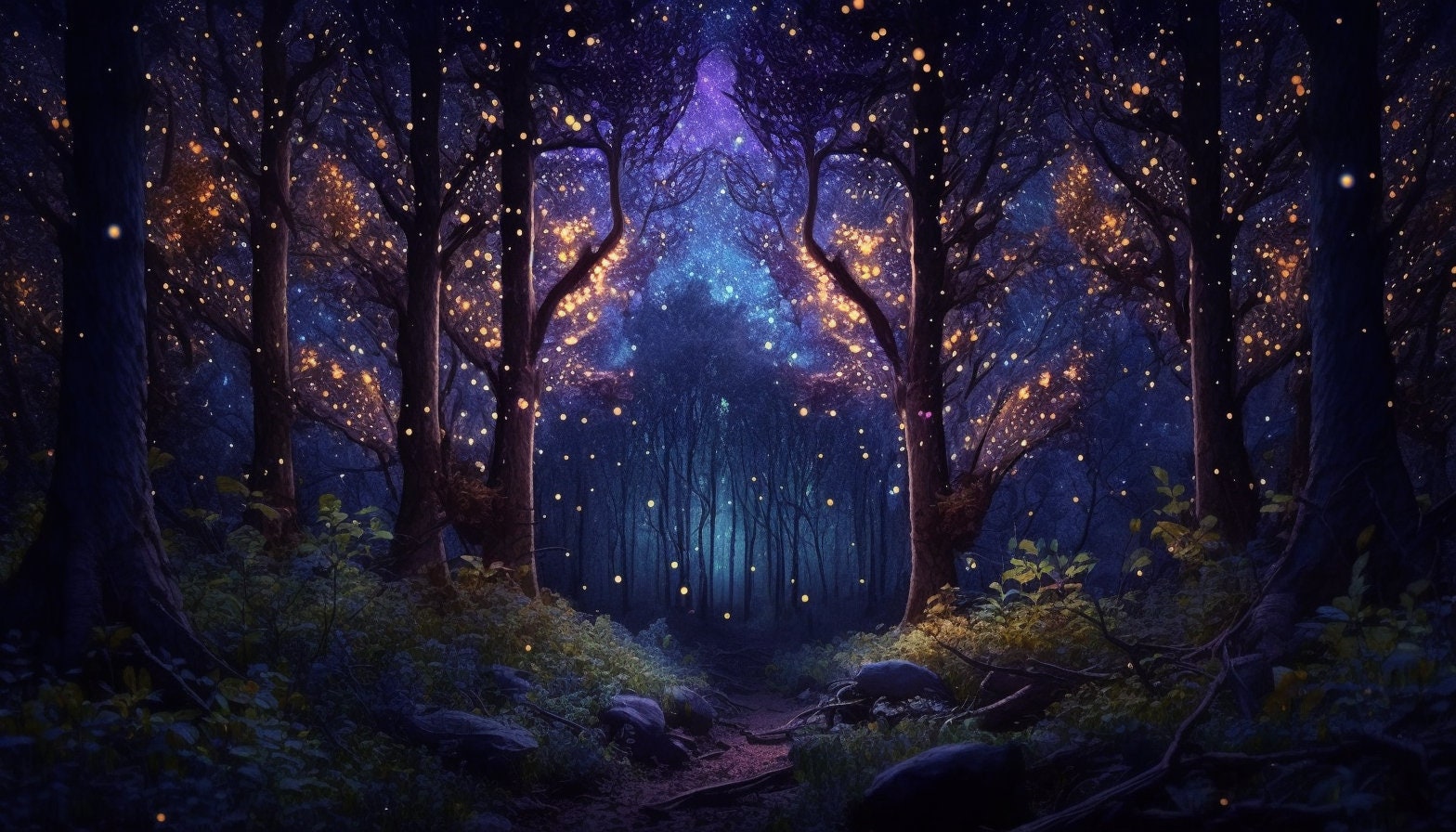The fantasy illustration depicts a mystical forest bathed in a deep, enchanting blue light. The scene is shrouded in a twilight ambiance, giving it a magical and otherworldly feel. In the foreground, a clear path winds through the forest, flanked by scattered rocks and lush shrubs, guiding the viewer's eye deeper into the scene. Midway through the forest, several trees are adorned with countless shimmering golden lights, reminiscent of magical fireflies or glowing pollen drifting through the air, casting a soft, ethereal illumination. Further in the distance, the forest grows denser and darker, with silhouettes of trees creating a sense of depth and mystery. The interplay of light and shadow paints a captivating and serene fantasy landscape, inviting the viewer to imagine the wonders that lie beyond.